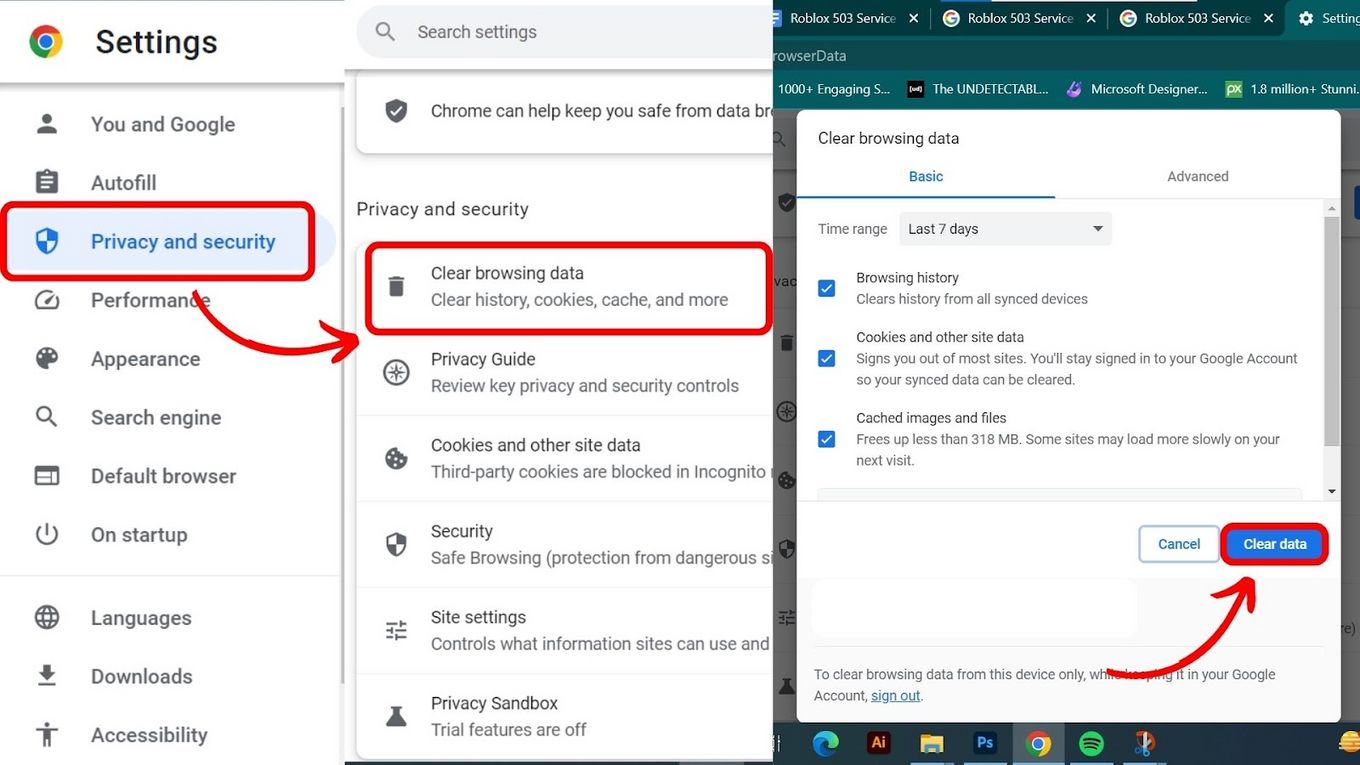The image depicts the "Settings" menu in Google Chrome, featuring a predominantly white background with a multi-colored circular Google logo (comprising red, yellow, green, and blue elements) at the top. Below the logo, there are several setting categories listed on the left side: "Settings," "You and Google," "Autofill," "Privacy and Security," "Performance," "Appearance," "Search Engine," "Default Browser," "On Startup," "Languages," "Downloads," and "Accessibility."

"Privacy and Security" is highlighted in blue, making it distinct from the other categories, which are in black on a white background. This section is further emphasized with a blue background and blue font. A box, accented in red, encompasses this section and directs attention to the "Clear Browsing Data" option, which is further broken down into "Clear History," "Cookies," "Cache," and "More."

A pop-up window, mainly white, appears labeled "Clear Browsing Data" at the top. Within this window, there are checkmarks next to "Browsing History," "Cookies and Other Site Data," and "Cached Images and Files." Below these options is a prominent blue button labeled "Clear Data," enclosed in a red circle with a red arrow pointing to it.

This image serves as a guide, visually explaining the process of clearing browsing data and cache in Google Chrome. The predominant colors in this depiction are green, blue, red, yellow, and some brown.